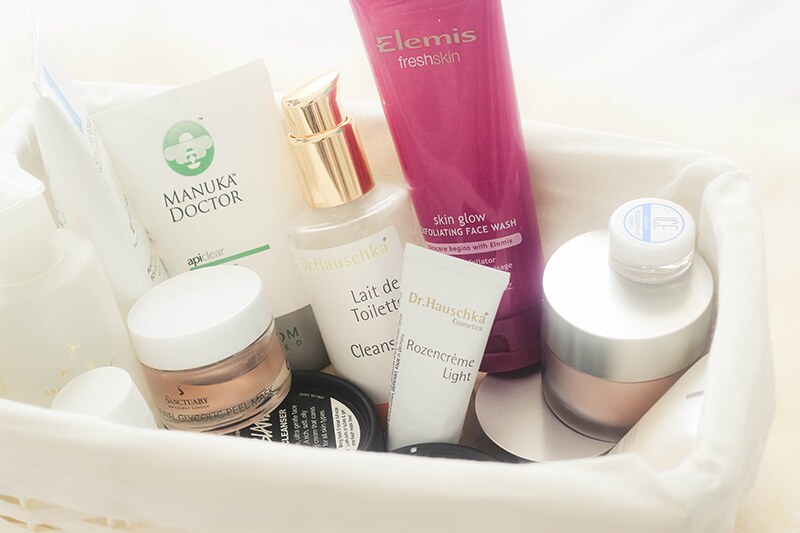This photograph showcases a white plastic basket, prominently positioned in the lower left corner of the image. The basket features a mesh design on its sides and is neatly lined with a white fabric liner. Inside the basket, an extensive collection of assorted makeup and skincare products is meticulously organized. The contents include items commonly found in a powder room or on a dressing table, ideal for use in front of a mirror.

In the basket, several recognizable brand names are visible, such as Manuka Doctor, EpiDeer, and Elemis. Specific products include the Elemis Fresh Skin Glow Exfoliating Face Wash and Dr. Poshka's skincare items. Among the assortment, there are various creams, including one labeled "Light Day Toilet," and a shallow jar bearing the label "Sanctuary," which is identified as a peel mask.

The assortment of items spans an array of container types, from pump dispensers and screw-top jars to flexible tubes, all neatly arranged within the lined basket. This composition is set against a pristine white background, emphasizing the clean and organized display of makeup and skincare products.